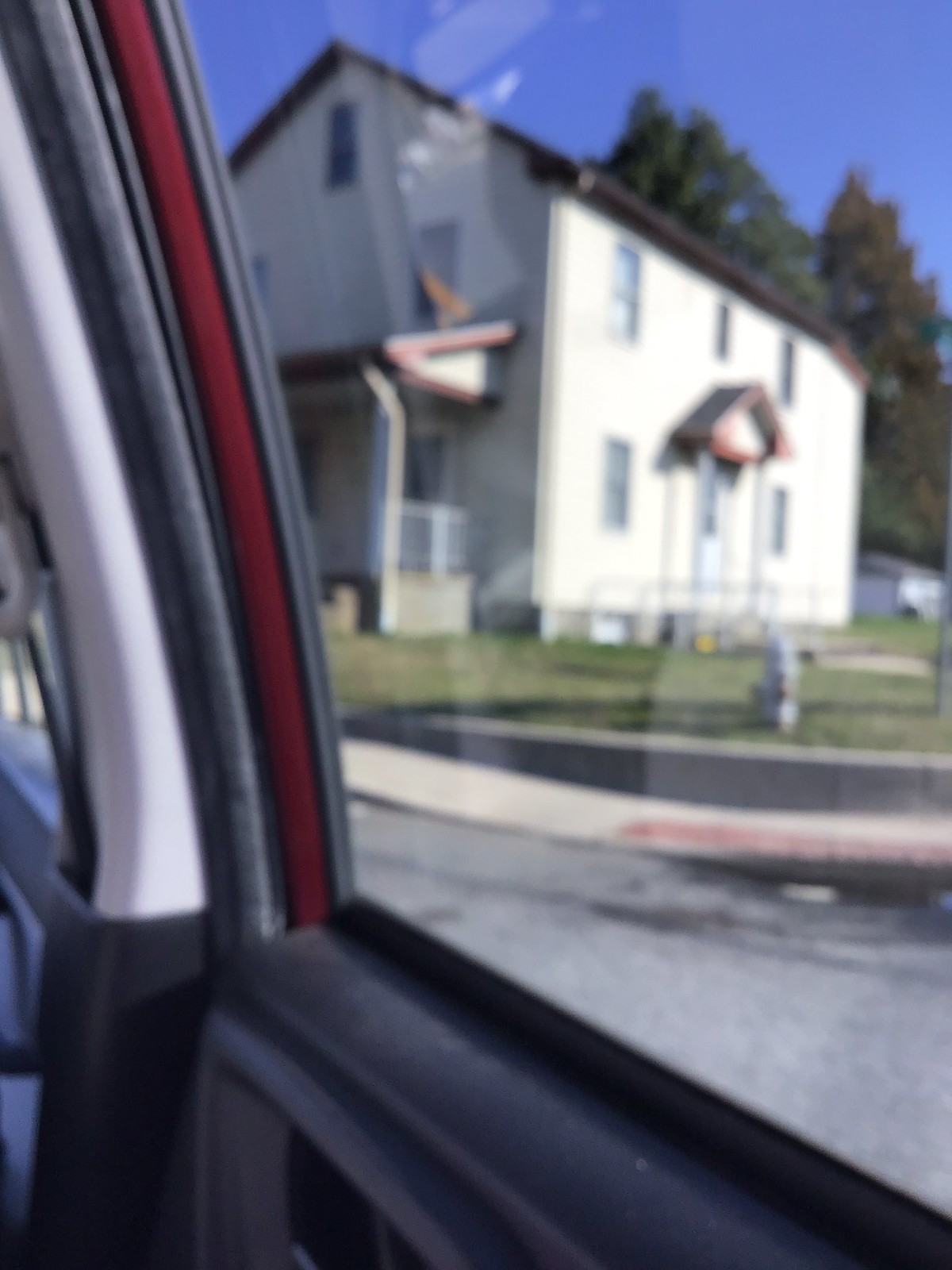Captured through the window of a moving vehicle, this somewhat blurry photograph showcases a cream-colored house against a backdrop of vivid blue sky. The interior frame of the image is tinged with dark charcoal gray from the vehicle's interior, while a hint of red marks the edge of the window. Beneath the moving vehicle, the asphalt street is a lighter shade of gray, leading to a light gray sidewalk that runs parallel. Adjacent to the sidewalk is a well-maintained, short lawn of light green grass.

The house features a symmetrical façade with five windows placed prominently at the front. At the center of the house, a large white door is accompanied by a modest overhang. The house is capped with a stark black roof, adding contrast to the cream-colored walls. Behind the house, evergreen trees rise, adding depth and greenery to the scene. The clear, vivid blue sky has no clouds, providing a serene and picturesque backdrop.